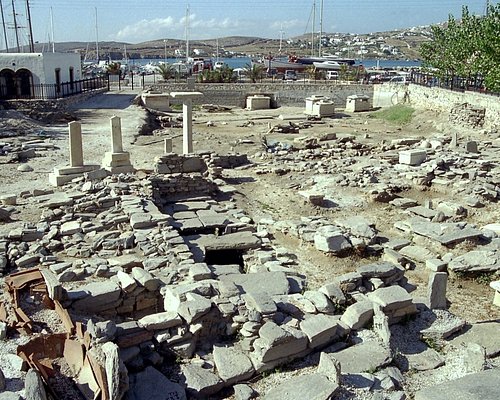The image depicts an archaeological dig site or ruins situated on the coast of an ocean or lake. It features meticulously cut stone slabs that are largely in disrepair, scattered across the area in what appears to be a graveyard or former buildings' remnants. Among the rubble, there are two or three tall, skinny monument-like stones standing erect. The site is enclosed by a stone wall, and there is random metallic debris strewn about. In the background, several boats are docked on the water, which is framed by low hills or mounds and some possibly inhabited houses. The top left corner shows a dilapidated building, while the top right is dotted with trees and foliage, adding a touch of green to an otherwise predominantly beige and broken landscape.